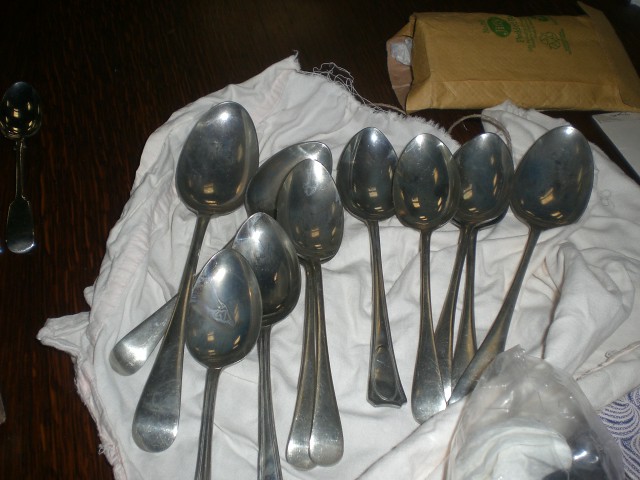This photograph captures a variety of silver tablespoons, mostly vintage and larger than average, scattered in a somewhat horizontal array atop a white, frayed cloth that appears to be on a wooden table. There are ten spoons, with most facing upwards, though a few appear to be facing down. One spoon is noticeably placed alone at the top left, directly on the wooden surface. Accompanying the spoons is a padded manila envelope, possibly their delivery container, positioned at the top of the image. There is a clear plastic bag in the lower right corner, resting on a design of blue and white beneath the cloth. The photograph was taken with a flash, indicated by the reflections seen on the spoons.